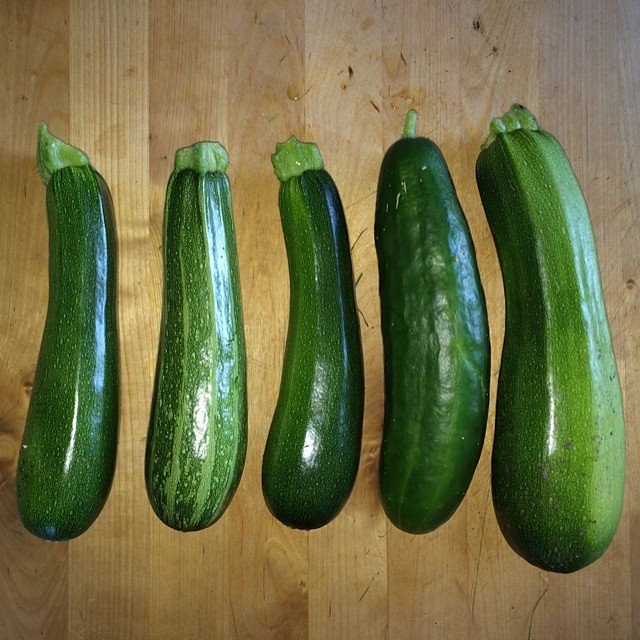This is a detailed close-up photograph capturing five zucchinis arranged in a row on a well-worn butcher block-style cutting board. The zucchinis are neatly ordered by size, from the smallest on the left to the largest on the far right. Notably, the fourth zucchini closely resembles a cucumber, with a distinct thinner and lighter stem, suggesting it might have been mistakenly included in the lineup. The zucchinis display a variety of green hues and patterns, with some showcasing glossy, smooth textures that reflect light either from a flash or natural sunlight. The cutting board itself bears the marks and stains of previous use, giving it a seasoned and utilitarian appearance. Additionally, small scuffs, black stains, and traces of moisture add to the rustic, everyday kitchen atmosphere depicted in the image.